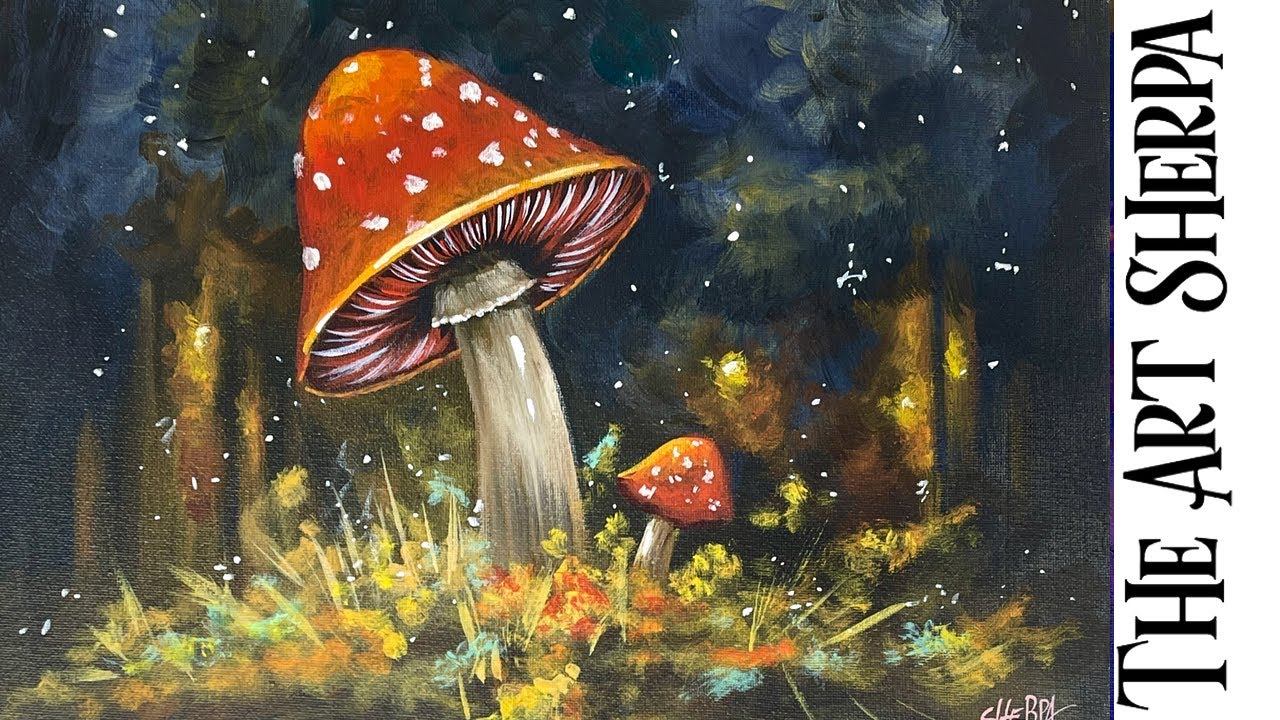This vivid artwork, potentially an expertly painted or digitally created piece, features prominently a large, bulbous mushroom with an orangish-red cap adorned with white spots. The mushroom’s stem is a beige-yellow hue, and a smaller mushroom sharing the same color scheme nestles to its right. The background is dark and atmospheric, appearing almost nebulous, with swirling shades of black, gray, and bursts of purples, oranges, and yellows that give a cloudy, even fiery impression. The ground from which the mushrooms emerge is alive with a mix of yellow, green, and darker hues, with paintbrush-like strokes giving a textured, vibrant effect. Notably, the right side of the painting features bold, sideways black text reading “The Art Sherpa,” likely indicating the creator. White flecks scattered throughout add a dynamic, starry quality to this captivating scene.